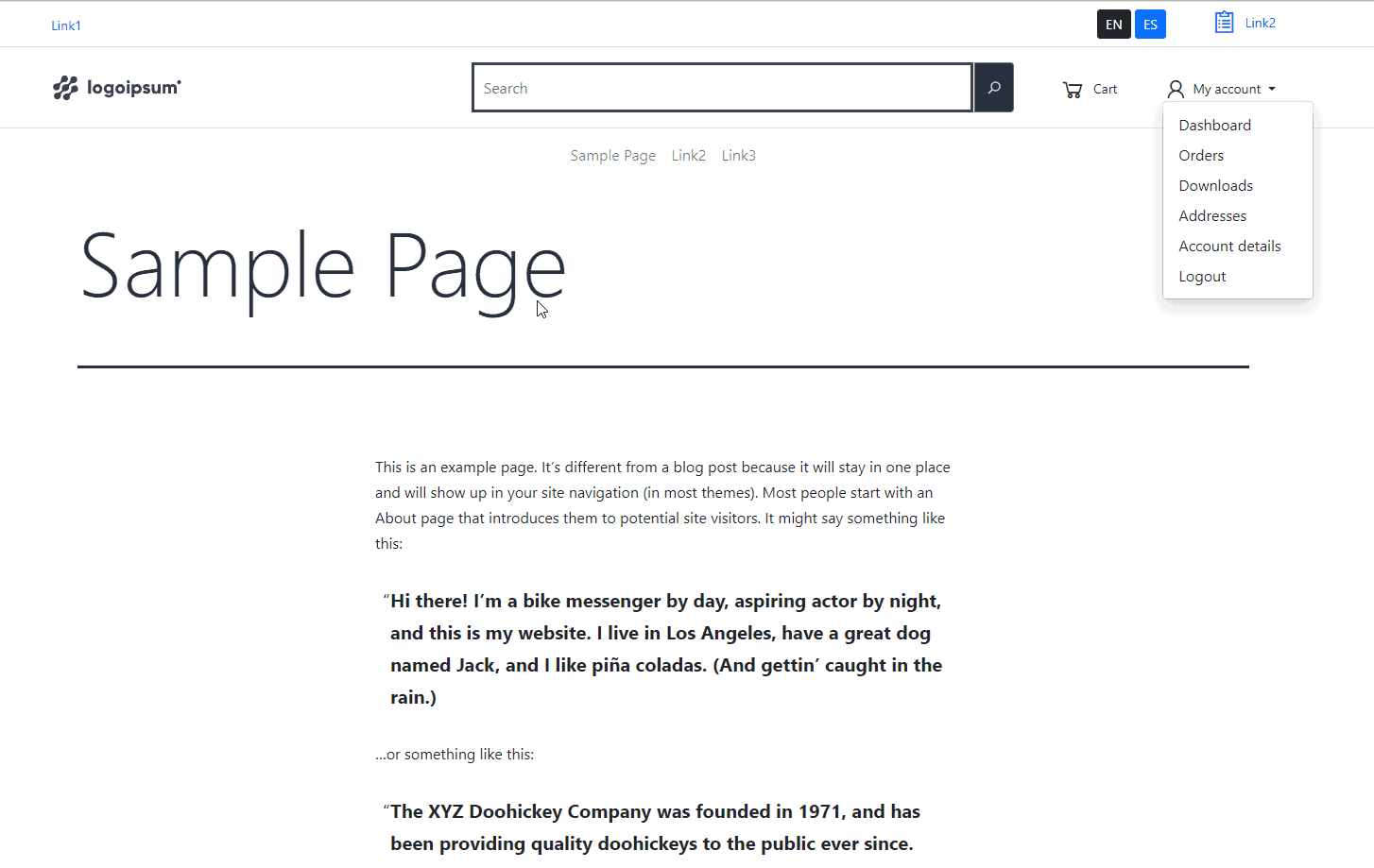At the top of the image, there is a very faint gray border. In the top left corner, in blue text, it says "link one" with no space between the words and number. To the top right, there are two adjacent squares; the left square is dark gray with the white text "EN" for English, and the right square is blue with the white text "ES" for Español. Further to the right, there is a blue clipboard icon followed by the blue text "link two," again with no spaces in between.

Below this section, there is an even fainter gray border. On the left side, there is a logo comprised of two connected dots, then three connected dots, and another two connected dots beneath them, all in gray. Below the logo, it reads "L-O-G-O-I-P-S-U-M" with a registered or trademark symbol in the upper right corner.

Next to the logo, there is a search area with a light gray text field that says "search." This text field is bordered by a dark gray line. Adjacent to the search field, there is a small white space, followed by a dark gray square containing a white magnifying glass icon angled towards the top right.

To the right of the search area, there is a gray shopping cart icon with the text "cart" next to it. Further right, there is a silhouette of a person accompanied by the text "my account" and a downward-pointing arrowhead indicating a drop-down menu. The drop-down menu is open and contains gray options: "dashboard," "orders," "downloads," "addresses," "account details," and "log out." The menu has a shadowy border around the bottom, left, and right sides to create a 3D effect.

Finally, towards the left in dark bluish-black text, it says "sample page." A cursor is positioned at the bottom left of the "E" in "sample page."